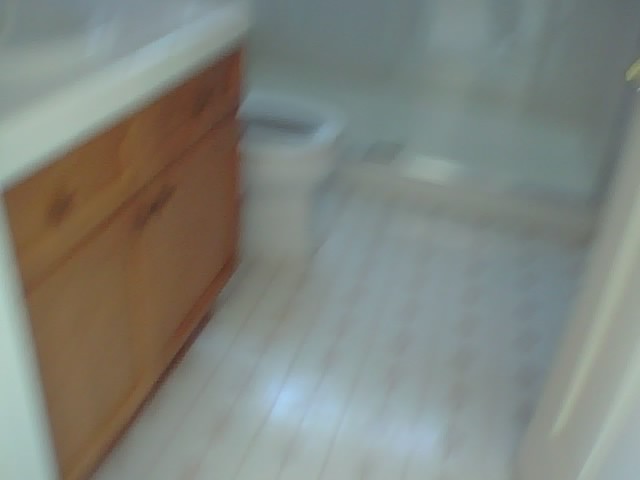This image depicts a small and blurred bathroom, making it challenging to discern specific details. Despite the lack of clarity, several elements are identifiable. On the left, there is a light wood vanity with dual cabinets that open on either side and possibly two shelves. It has a white countertop, which likely houses a basin and faucet. Adjacent to the vanity is the bowl of a white toilet, mostly visible from the pedestal to the seat. The bathroom floor is tiled or possibly linoleum with a faint pinkish design that is difficult to make out due to the blurriness. Further into the room, there appears to be an open shower area, likely featuring a glass door or a transparent shower curtain. The room's muted colors suggest a light and airy space, characteristic of a small, simple bathroom in an older home.